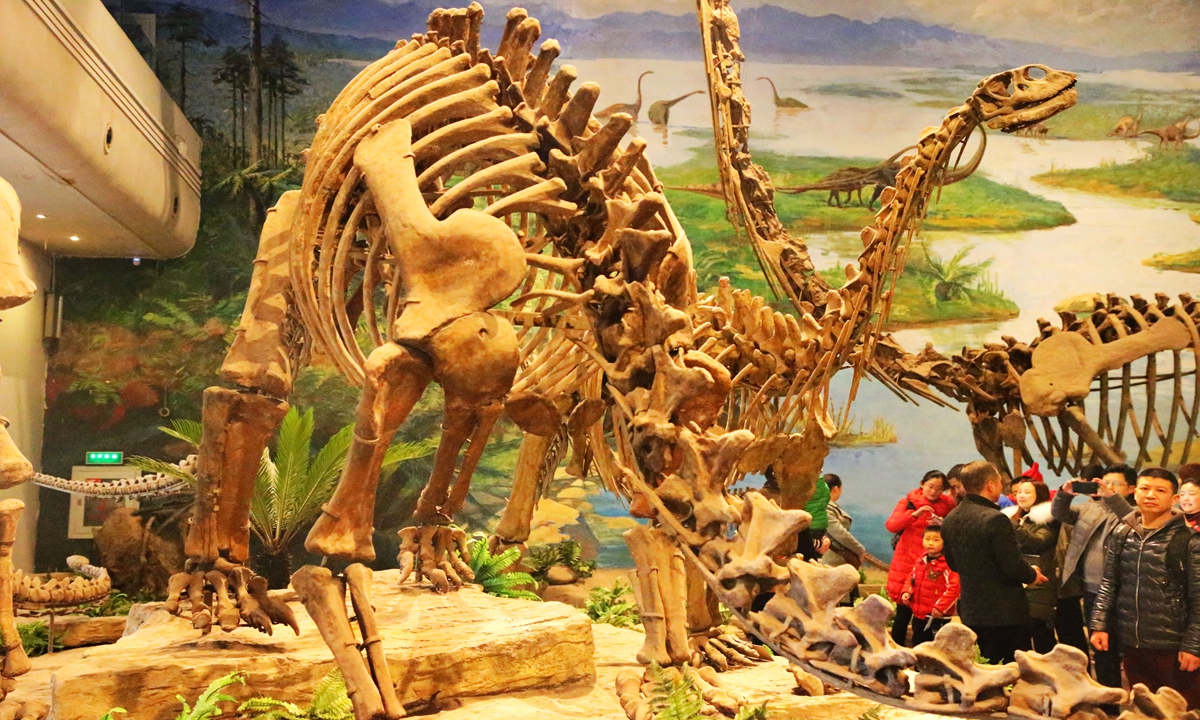The image captures a detailed photograph of a museum interior where a group of approximately 20 tourists, including some children, are observing an exhibit featuring large dinosaur skeletons. Central to the scene is a museum guide engaging the visitors, who appear to be of diverse backgrounds, possibly of Asian descent. Dominating the foreground, two impressive long-necked dinosaur skeletons, their tannish bones prominently displayed, are set on rock-like platforms. One skeleton, fully formed with an elongated tail, spine, and high-held head with large eye sockets, gestures toward its life-like depiction. Surrounding the skeletal remains is a recreated prehistoric habitat, adorned with ferns, rocks, and other flora, providing context to the exhibit. The backdrop reveals an expansive hand-painted mural with vibrant shades of green, brown, and blue, depicting a wetland scene complete with dinosaurs in an ancient aquatic environment. The detailing includes a wandering blue river and green dinosaurs seemingly foraging, adding depth and realism to the museum's portrayal of prehistoric life. To the left, a plain white wall is accentuated by a couple of yellow hanging lights and an exit sign, highlighting the meticulous design elements of the exhibit.